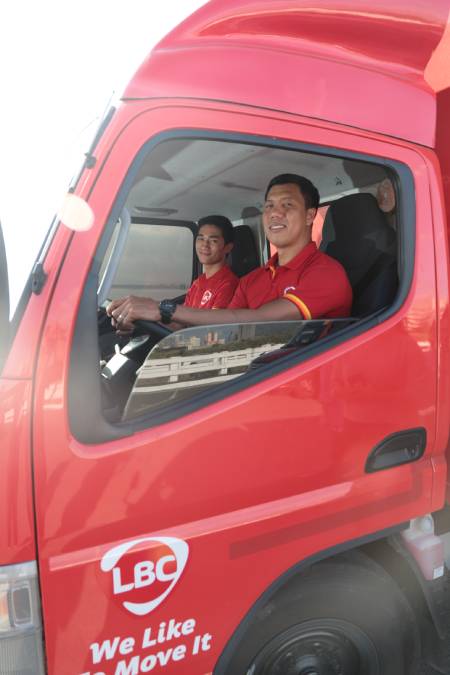In this detailed outdoor daytime photograph, two Asian men are seen sitting in the cab of a red semi-truck, both wearing red polo shirts with the LBC logo, accentuated by yellow and orange stripes on the sleeves. The driver, sporting a black watch, and the younger man seated behind him, both smile at the camera. The truck features distinctly black tires, a black door handle, and contains a reflective window, partially rolled down. The truck exterior is marked with the text "LBC" in white, positioned within a white circle, accompanied by the phrase "we like to move it" below. The interior is a combination of white and gray, with gray seats and a black steering wheel that has silver accents. The background reveals a grey sky and a white structure reflected in the truck's window. The front of the truck is highlighted with white light fixtures and some orange accents.